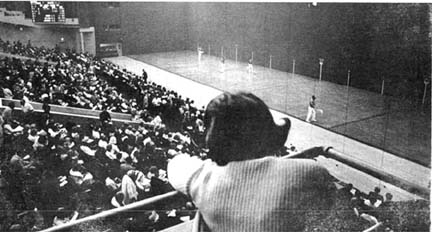This black-and-white photograph, likely from the 1950s or 1960s, depicts a bustling scene within a large, blurred auditorium or sports arena. In the foreground, a woman with a black bob haircut and wearing a ribbed white sweater prominently stands out, seemingly directing her attention or pointing towards something amidst the crowd—a crowd that fills the bleachers with indistinct, shadowy figures. The spectators, somewhat blurred and indistinct, are fixated on simultaneous on-court action resembling a game involving a ball and scoops, possibly jai alai or tennis. The photograph offers a nostalgic view, characterized by its lack of sharpness and abundant shades of gray, capturing the fervent atmosphere of the games being watched.